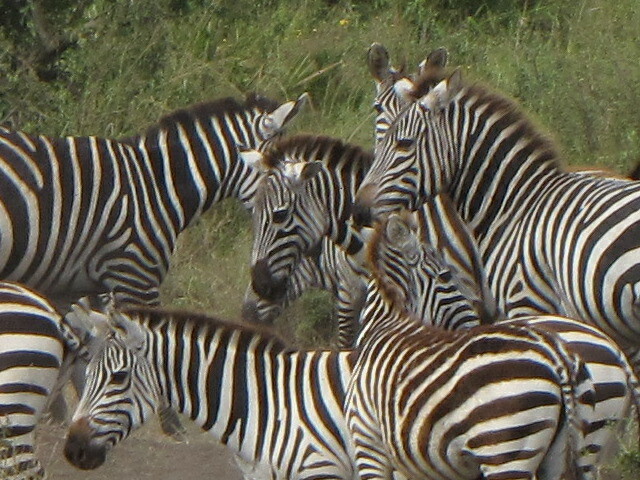The photograph captures a small group of zebras, appearing almost identical with their distinctive white bodies adorned with black stripes, and short black or gray manes. There are five zebras clearly visible, with a few others partially cut off by the frame's edges. Each has black eyes, black noses, and white ears. The zebras are positioned at various angles, with some facing different directions. One zebra in the front turns its head to the right, adding a dynamic touch to the scene, while others seem to look downward or straight ahead. A peculiar lump is seen dangling from the neck of one zebra. The entire group stands on a grassy field with long grass, dotted with small yellow flowers and a dirt path beneath them. The blurred background accentuates the focus on the zebras, making their intricate patterns and features the centerpiece of the image.